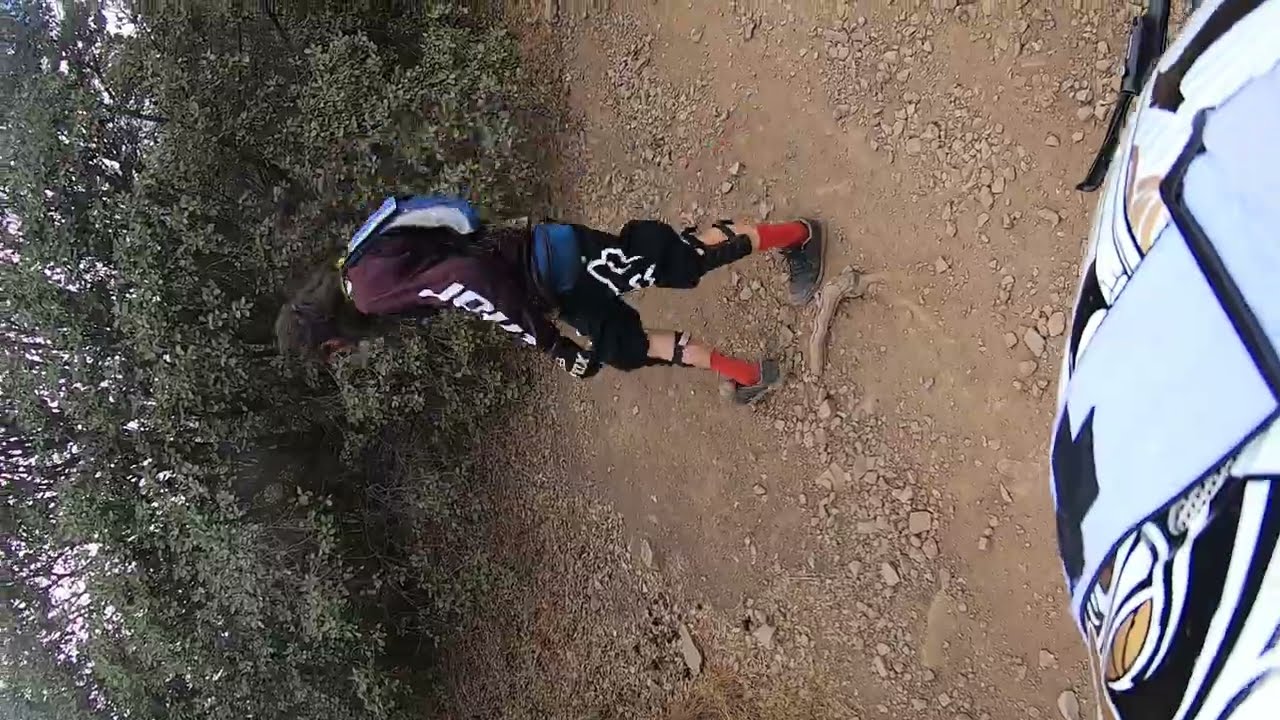The image shows an outdoor scene oriented incorrectly, appearing sideways but initially taken in portrait mode. Central to the image is a person, potentially a man, dressed in what looks like motocross or paintball gear. He wears black shoes with tall red socks, black shin guards on bare legs, black shorts sporting a white fox design on the left leg, a blue fanny pack, and a long sleeve burgundy shirt with white font on the sleeves. His hands are covered with black gloves, and he carries a white and blue backpack. 

The person is walking along a dirt path scattered with stones and little rocks, surrounded by a lush backdrop of trees and shrubs with dark green leaves. Closest to the camera, there is another person partially hidden, wearing white clothes adorned with black designs. In the lower portion of the photo, which appears on the right due to the image rotation, there is a blue, white, and black item, possibly a tent or bag, with some logo on it. The forested area and the dirt path suggest a woodsy, outdoor environment.